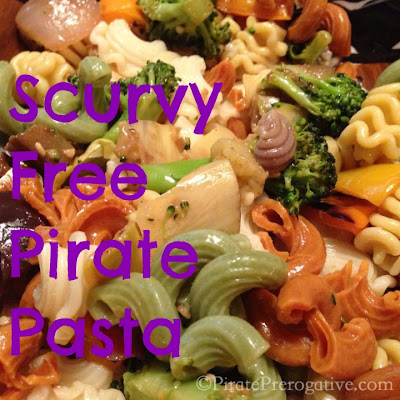This horizontally-aligned, somewhat blurry photograph showcases a vibrant, close-up shot of a colorful pasta and vegetable medley. The image features various types of curved pasta in diverse hues—orange, green, white, and possibly other shades—suggesting ingredients like carrots and broccoli, or simply playful coloring. Interspersed among the pasta are small, blanched pieces of broccoli, and what appears to be shiny, wet items that could be additional pasta or seafood. The dish also includes scattered pieces of red onion. Overlaid prominently in vivid purple text, each word stacked vertically and left-aligned, are the words "Scurvy Free Pirate Pasta," with only the first letters capitalized. The photograph is marked with a copyright notice at the bottom, indicating "pirate prerogative dot com," in mostly lowercase, somewhat translucent white letters.